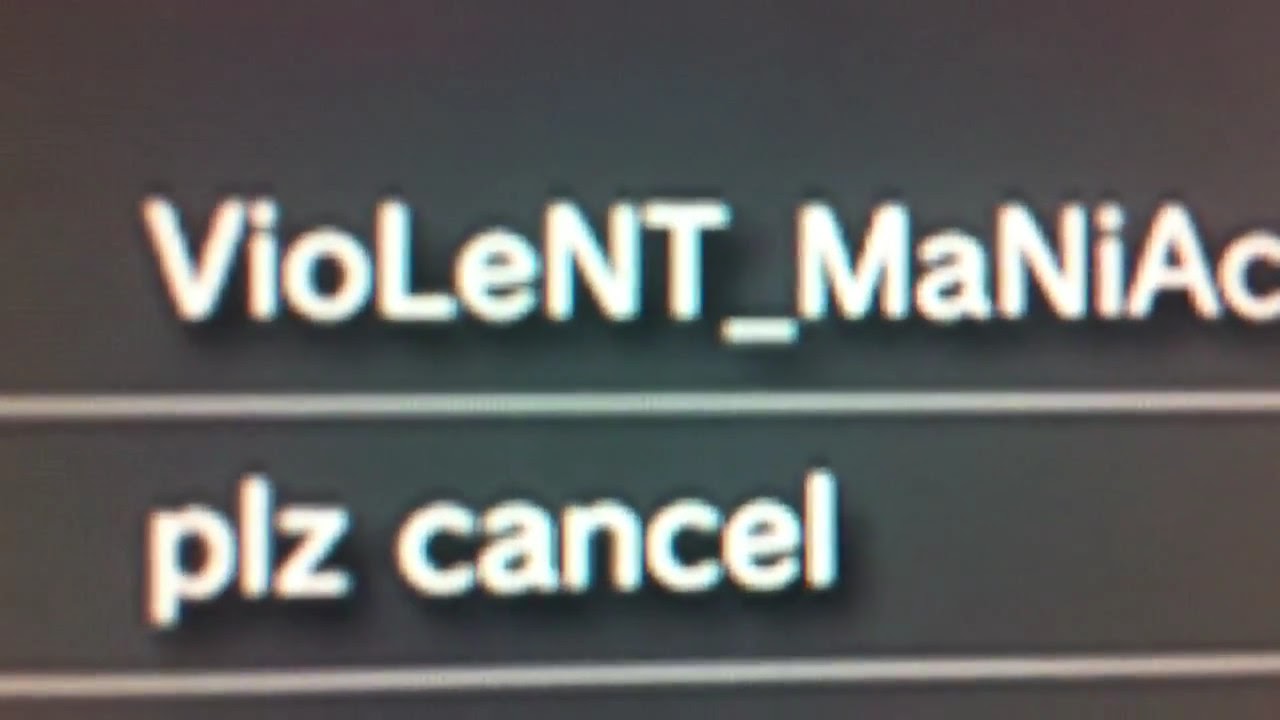The image displays a dark gray rectangular background featuring a series of white lines and text that resemble a computer screen. Centered within the frame, the text is divided into two sections by a horizontal white line. Above the line, in a combination of uppercase and lowercase white letters, the text reads "VIOLENT_MANlAC" with the specific capitalization: "V,I,O," (lowercase), "L,E,N,T," (uppercase), "_," (underscore), "M," (uppercase), "A," (lowercase), "N," (uppercase), "I," (lowercase), "A," (uppercase), "C." Below the line, the text "PLZ CANCEL" is displayed, also in white lowercase letters, with another uninterrupted horizontal white line beneath it. The image is devoid of other objects, giving it a stark and minimalistic appearance. The overall composition suggests a screen capture, possibly of a username or command prompt, presented in a simple and direct format.